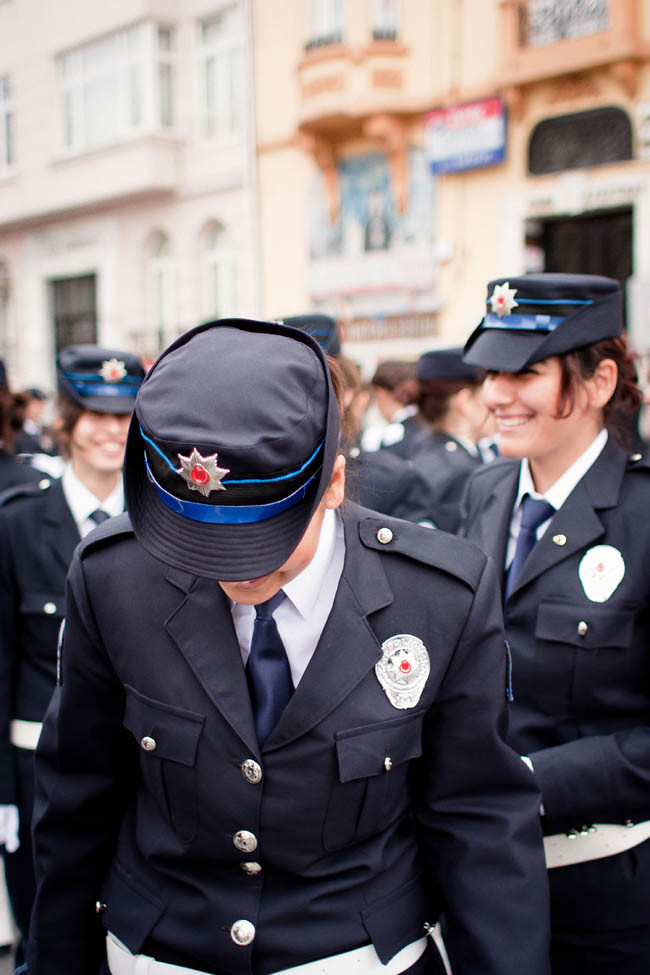A large group of young women in dark navy blue uniforms, complete with silver buttons and insignia, congregate outside in front of two buildings. They are part of an armed forces or military unit, and their attire includes navy hats adorned with light blue ribbons and a prominent golden star with a red center. The women are dressed in black overcoats with white shirts, blue ties, white belts, and white gloves. The uniform is also detailed with silver buttons along the lapels and chest pockets, each adorned with a badge displaying a white star and red center. In the front of the group, three officers are positioned close enough to discern facial features, although the central officer has her head tilted downward, partially obscuring her face. This officer, though her expression is somewhat obscured, appears to be smiling, as do many of those who face the camera. Behind them, two buildings are visible: the left structure is a peach color, and the right is yellow with darker ochre accents around the second-story windows. Both buildings have distinctive round doors, contributing to the scene's architectural setting.